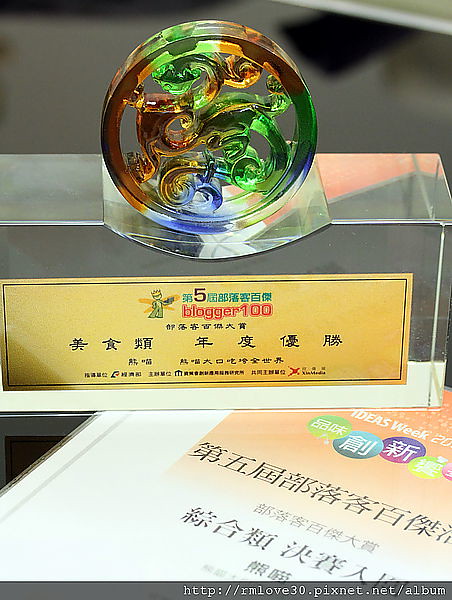This photograph features an award prominently displayed on a table. The central element of the image is a clear, rectangular glass prism with a curved top surface, upon which rests a circular glass object. The circular object is intricately designed with a multicolored pattern in green, blue, and orange, featuring a dragon carving at its center. This multicolored circle adds a vivid focal point to the award.

Attached to the front of the rectangular prism is a gold label with red text that reads "Blogger 100," accompanied by numerous Chinese characters. The label is yellow, enhancing the contrast with the red lettering. Positioned below the glass prism is a piece of white paper that contains a mix of Asian characters in black and white text. The paper includes an orange rectangular section at the top labeled "Deals Week" and features various colored bubbles—green, light blue, purple, light green, and pink—each containing white Chinese characters. Additionally, there are four lines of black Chinese characters located further down the sheet.

The award, with its intricate and culturally rich elements, appears to recognize a significant achievement in blogging, as denoted by the "Blogger 100" inscription.